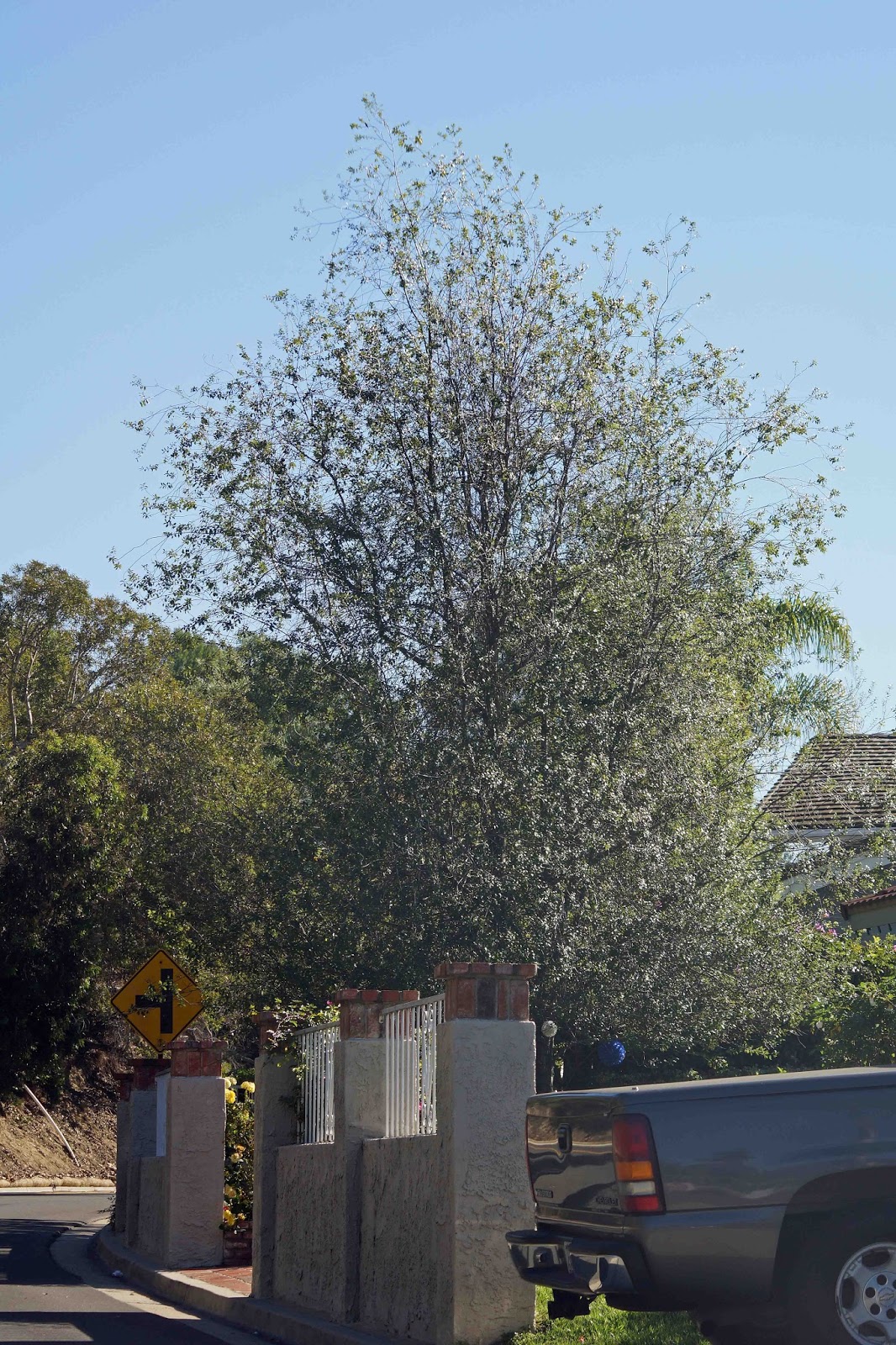The photo, taken on a sunny day with a mostly clear blue sky, features a large, green tree prominently in the center, likely a young oak, given its distinctive leaves. The tree is situated on a curb outside a house, which suggests it is in a residential neighborhood. The curb is lined with a brick path and several short stone columns, adding a decorative element to the area. On the bottom right of the image, there's a dark grey pickup truck, partially visible, while the paved road on the bottom left curves around a bend. A yellow diamond-shaped street sign featuring a black, downward arrow with a leftward bend is located on the left side, and additional trees can be seen in the background, contributing to the overall lushness of the scene.